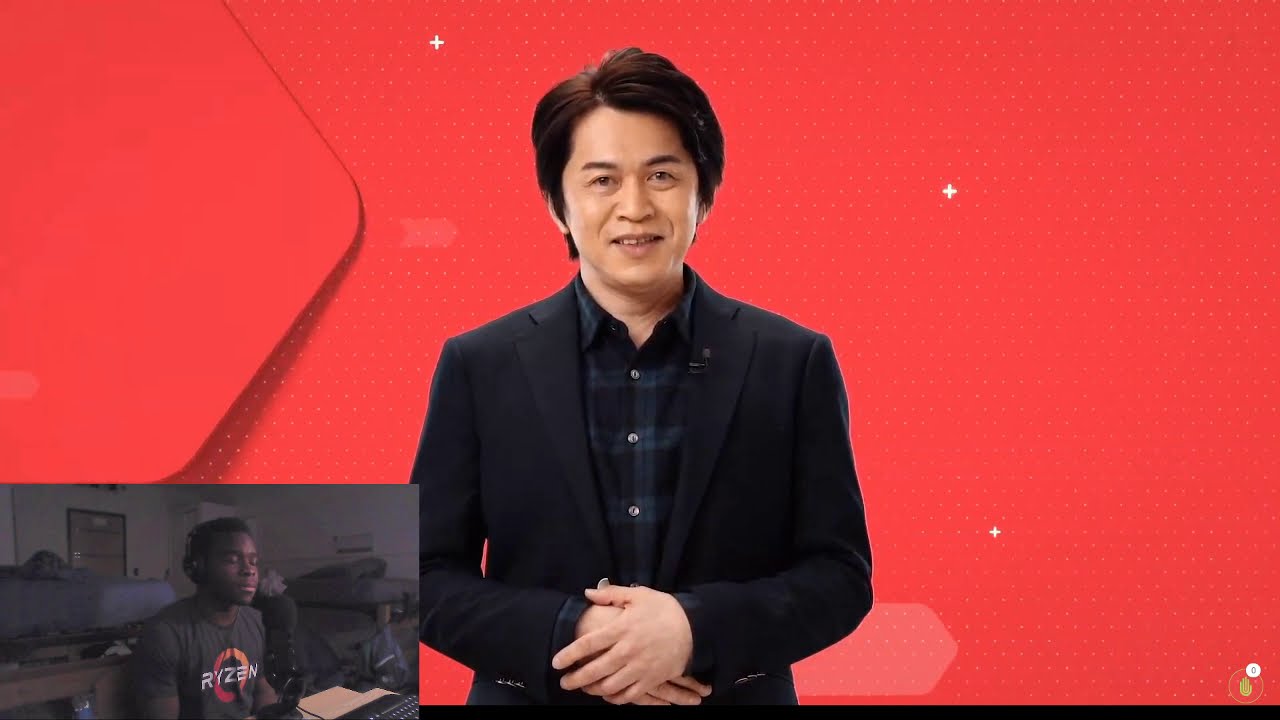The image depicts an Asian man with short black hair, standing with his hands gently folded at his waist. He is smiling warmly at the camera, wearing a dark plaid button-down shirt under a black blazer, accessorized with a small microphone on his collar. The background is predominantly red, transitioning to lighter pink near the bottom, embellished with white dots and plus sign designs. In the lower left-hand corner, there is an inset box showing a young African-American man seated at a computer. His eyes are closed, and he is wearing headphones and a black shirt that reads "Verizon" with a yellowish-orange circle in the center. He appears to be in a bedroom, speaking into a large microphone positioned in front of him.